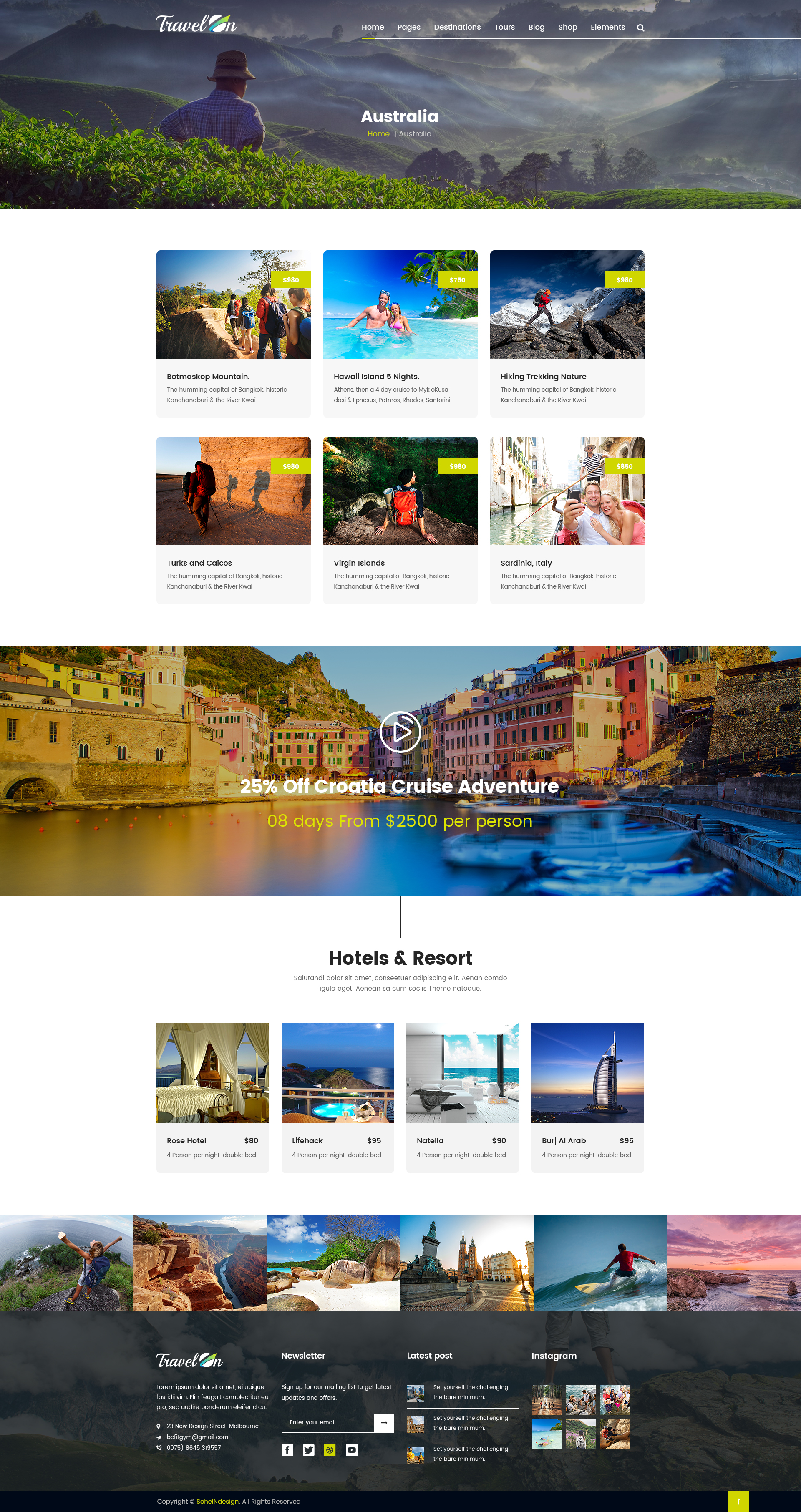The image is a collage divided into various sections, each highlighting different travel destinations and promotions.

At the top section, a horizontal rectangular frame depicts an outdoor scene. Central to this scene is a man facing away from the viewer, slightly left of center, donned in a hat. The upper left corner showcases lush grass and bushes, while the background features a range of majestic mountains. The word "Australia" is prominently displayed in bold white font across the middle. To the left of the text, there is a name or title that is indistinct, accompanied by menu items that are too small to decipher.

Below this, another horizontal section presents a row of three pictures, each accompanied by a brief description in black font. These images depict various travel locations, some featuring tourists engaged in activities. Beneath this row, a second set of three similarly described images continues the display, reinforcing the theme of travel destinations and experiences.

Next is a sizable horizontal rectangular image, akin to the initial one labeled "Australia." This scene is dominated by urban buildings in the background and a body of water or river running through the center, dotted with boats on the right-hand side. Superimposed in white font across the middle is the phrase "25% off Croatia Cruise Adventure." Below, in yellow font, it reads "8 days from $2,500 per person." A thin black horizontal line separates this section from the next.

Continuing downward, a subsequent horizontal segment features the heading "Hotels and Resorts" in black font on a white background. This area is segmented into four images, each lined up horizontally and annotated with additional details underneath.

At the very bottom, a black rectangular horizontal section offers further information. Positioned atop this dark background are six images, each portraying various travel sites and experiences, enhancing the rich tapestry of travel options depicted in the image.